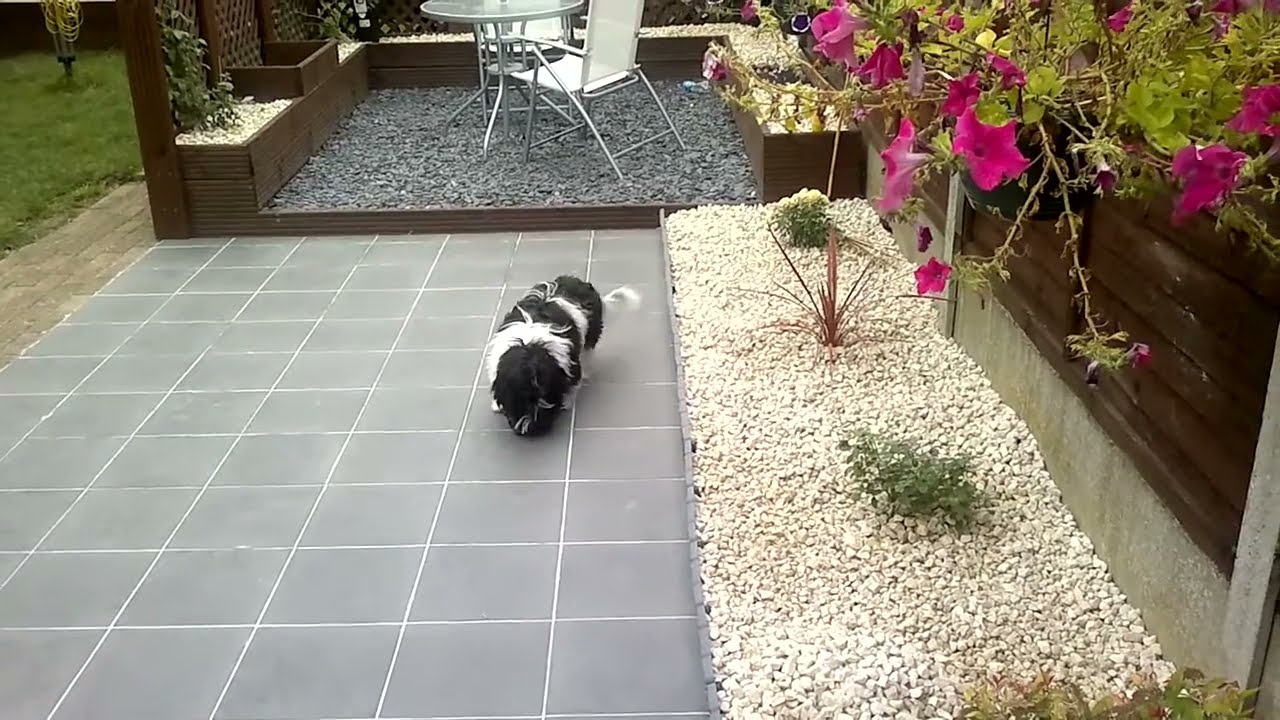The image showcases a meticulously designed backyard of a house with various distinct features. At the center is a small, furry black-and-white dog with alternating stripes of black and white fur. The dog stands on a paved gray tile floor with white mortar between the tiles. To the left, there is a section with white gravel containing wet flowers and a couple of small green plants. At the far end of the backyard, there is a cozy patio area featuring a round glass table and two large white chairs, surrounded by dark brown wooden planters filled with white rocks and vibrant plants. Surrounding this patio area are green vine plants climbing the wooden walls. On the top left corner of the image, you can spot a patch of grass with another green plant growing in it. Hanging above on the right side is a basket brimming with bright pink flowers, adding a splash of color to the scene. The backyard overall exudes a serene, well-maintained atmosphere with a combination of natural and thoughtfully arranged elements.